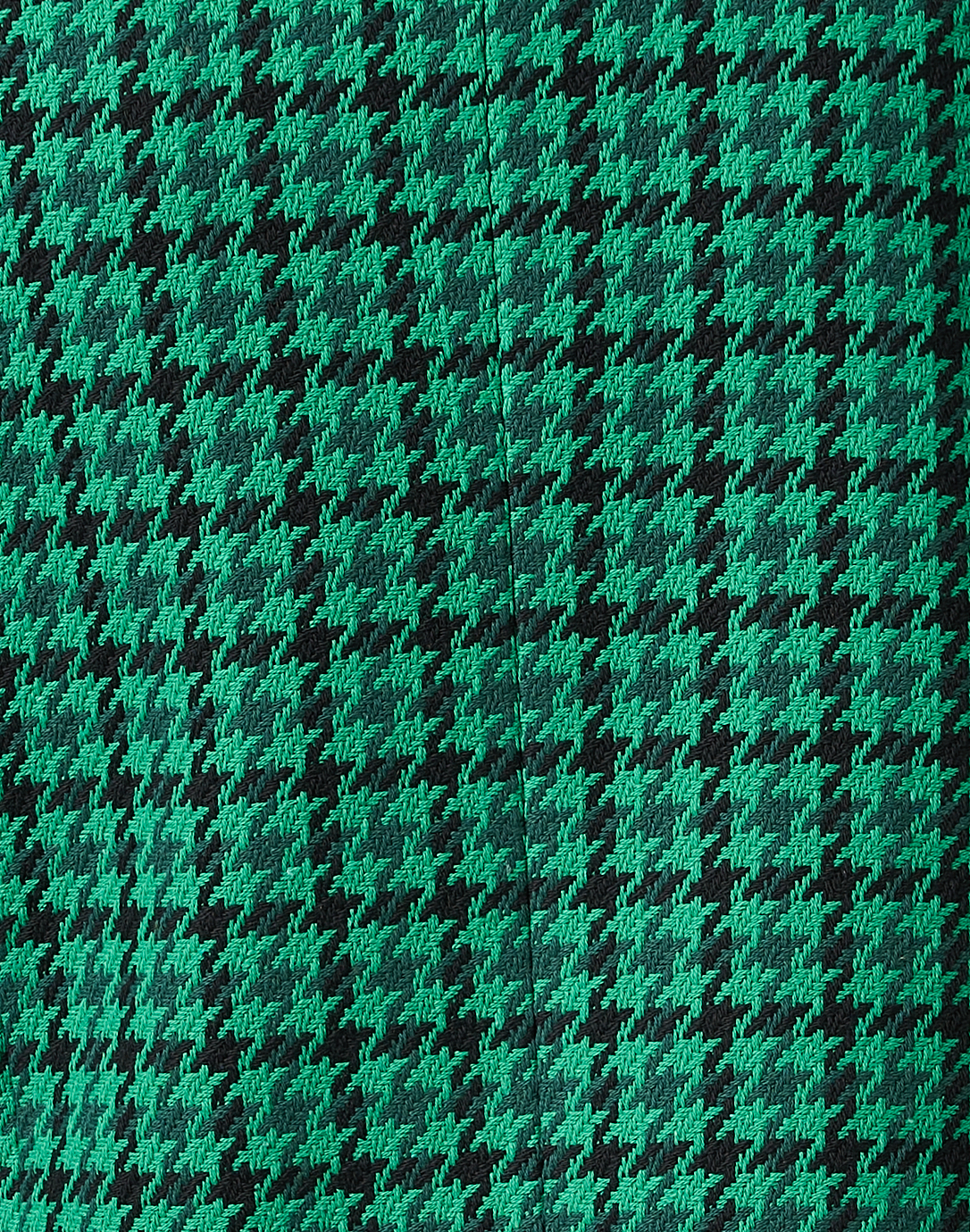The image is a close-up view of a fabric featuring a detailed pattern. The fabric is predominantly green, exhibiting light and dark shades interwoven with black. The design resembles a plaid or argyle pattern, frequently seen on jackets or furniture upholstery. A distinct seam runs down the middle, adding to the intricacy of the texture. The pattern contains elements that might resemble deformed lightning bolts or a symbolic, geometric motif, though it's not clearly identifiable. The close-up perspective emphasizes the woven, knit material and the square, latched-together stitching. The fabric's vibrant and complex design takes up the entire frame, leaving no background or context visible.